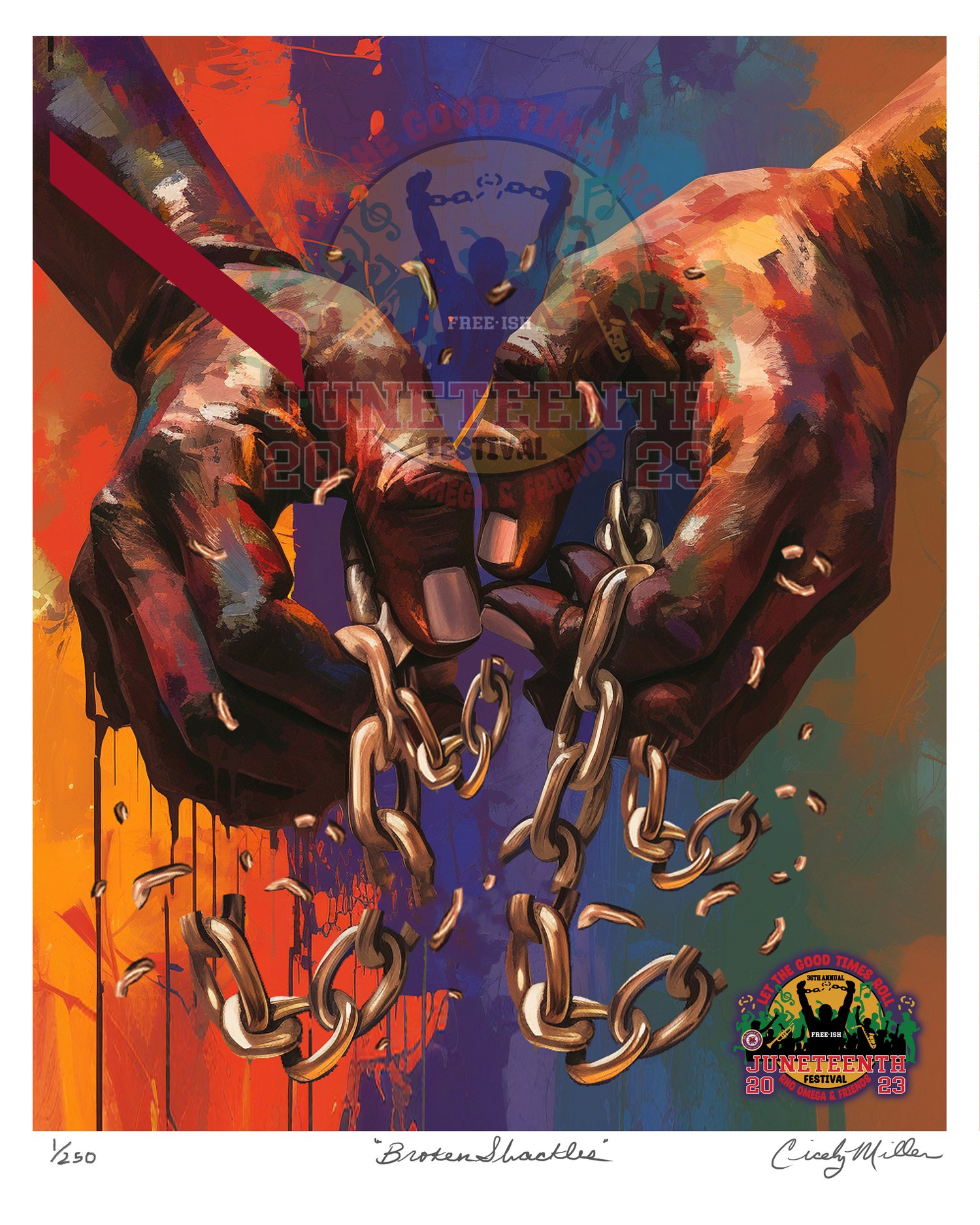The image is an art print titled "Broken Shackles" by Cicely Miller, numbered 1/250. The artwork features the detailed watercolor depiction of a black man's hands and wrists with golden chains, which are shown breaking apart within his fingers. The background is a vibrant blend of colors, transitioning from orange on the left, to purple in the middle, to teal, and then darker orange on the right. The print includes a white border around the edges, with a signature by the artist in the lower right corner. Below the main image, there's a logo and text highlighting the "Juneteenth 2023 Festival" with the phrase "Let the good times roll." A watermark with "Juneteenth" can also be seen at the top.